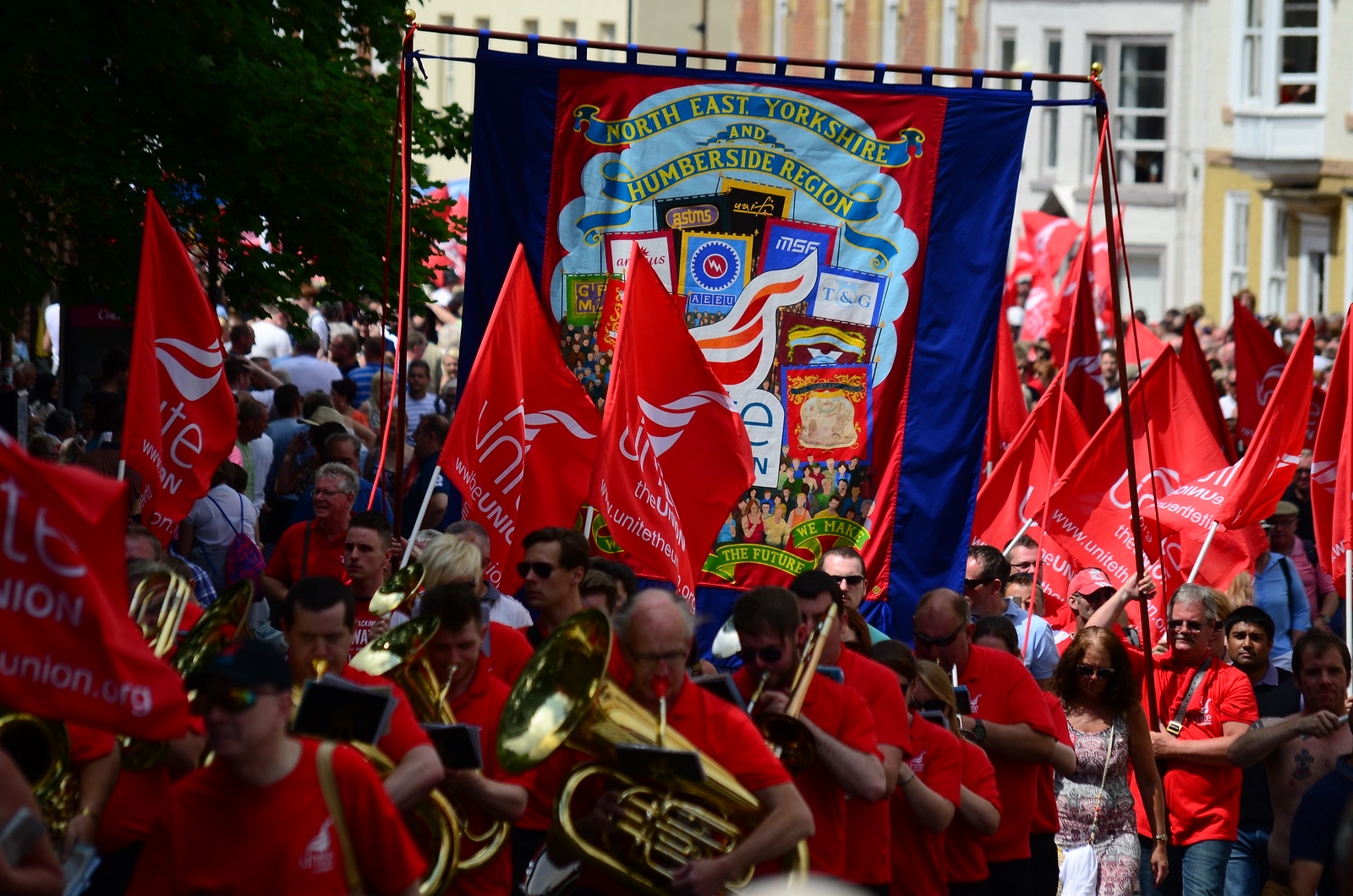In this vibrant outdoor photograph, we see an animated parade featuring participants from the Northeast Yorkshire and Humberside region. Central to the scene is a large banner carried aloft by two individuals, one on each side, which prominently displays the text "Northeast Yorkshire and Humberside region" along with the slogan "The Future We Make." The banner features a colorful mix of blue and red with various detailed illustrations of placards depicting smaller parades.

Predominantly, the parade boasts a spirited marching band, with members donned in red t-shirts. These musicians, captured mid-march and in lively motion, play an assortment of brass instruments including tubas and trumpets. The crowd surrounding the band is equally enthusiastic, many holding smaller red flags with a white insignia and partially visible text, appearing to say "WWW Unite the...".

The setting is outdoors with warm weather attire indicated by the short sleeves and summer clothing of the participants. Among the crowd, one man stands out in the bottom right corner, wearing only underwear. The scene captures the essence of the parade with the backdrop featuring a mix of urban and natural elements, such as green trees and a combination of white and beige buildings with visible windows, which add depth to the bustling atmosphere. The overall color palette is lively, dominated by reds, whites, blues, greens, and hints of yellow, reflecting the energetic and diverse nature of this regional celebration.